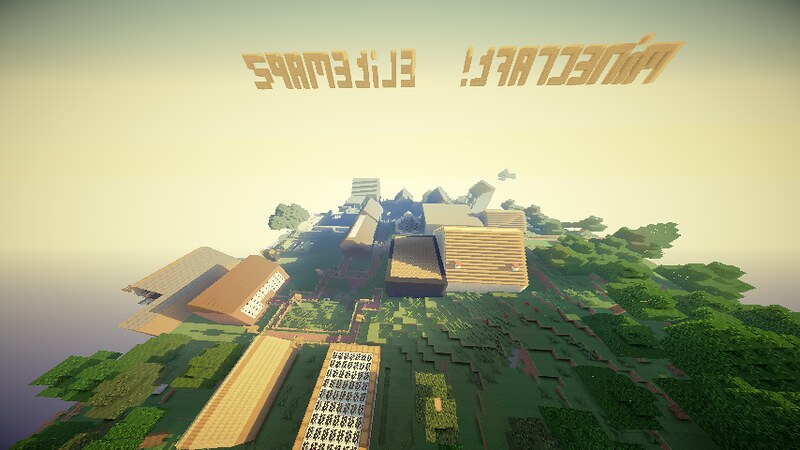This image showcases an overhead perspective of a digitally-rendered cityscape, likely featured in a computer game, video game, or animated film. At the top of the image, there is text written in an unfamiliar foreign language, and it appears mirrored, indicating we are seeing it from behind. The background is divided into three distinct color gradients: a dark blue or black sky at the top, transitioning to a vibrant yellow in the center, and then light blue at the bottom, which could possibly represent water. The town below is characterized by a vivid green landscape interspersed with a few trees and grassy areas. The design is noticeably angular and blocky, with clear, solid corners defining the terrain and structures. Within the town, there are approximately eight houses, the most prominent of which features a brown roof and a white facade. Other structures are present, but their identities are obscured by the simplistic and blocky art style.